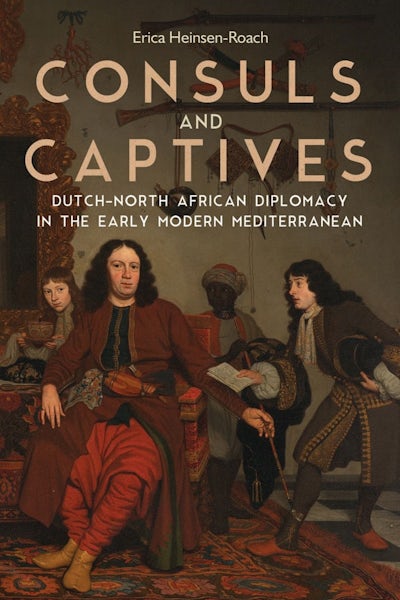The cover of the book "Consuls and Captives" by Erika Hansen Roach features a detailed painting set in a lavishly decorated room. At the top, the book's title is prominently displayed in large text, with the subtitle, "Dutch North African Diplomacy in the Early Modern Mediterranean," written below in smaller letters. Above the title, the author's name, Erika Hansen Roach, is presented in smaller text. The painting depicts a group portrait of four figures, three standing and one sitting, against a backdrop adorned with a mirror, rifles, and intricate ceremonial swords. The central figure, a Caucasian man in a red billowy robe and pants, sits on an ornate red chair. To his left, a young Caucasian man holds a decorated bowl, while directly behind the chair stands a dark-skinned man in a white robe and red cap. On the far right, another Caucasian man, dressed in a lavish brown robe and with long black hair, holds a hat and appears to be interacting with the seated gentleman. The painting's background has a white, tannish hue, reminiscent of the Renaissance period, and overall exudes an air of elegance and historical significance.